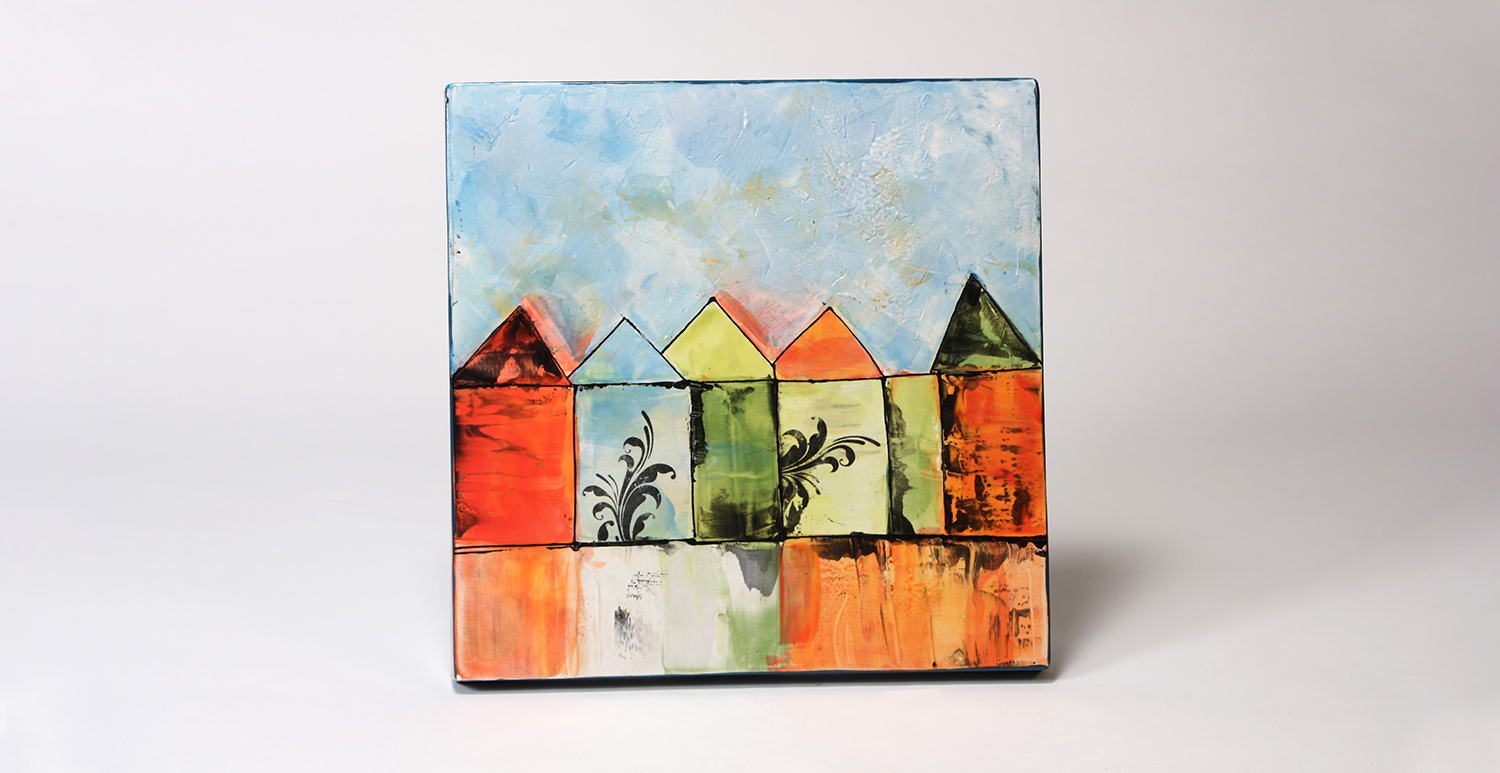The image features a small, square canvas painting set against a plain gray background with a prominent dark gray shadow cast to the bottom right, indicating a light source from the left. The painting itself is divided into two distinct sections. The upper part of the painting portrays a light blue sky with visible brushstrokes and white patches suggesting clouds. There are also hints of tan and reddish hues scattered within the sky. 

The bottom half depicts a series of six rectangular structures resembling houses, each topped with colorful triangular roofs. These houses vary in color: the leftmost house is red with a black and red roof; the next is light blue with a light blue and white roof and a leafy object in front; followed by a green house with a yellow roof, this one also has some black and blue streaks; then comes a yellow house with an orange roof; and finally, an orange house which has a black and green roof. Each house is accentuated by a dark green leaf-like shape in front of it.

Beneath the houses is a light brown area with a white center that gives the impression of a pathway or stream. The detailed and vibrant color palette of the painting contrasts with the minimalist gray background, drawing focus to the artwork itself.